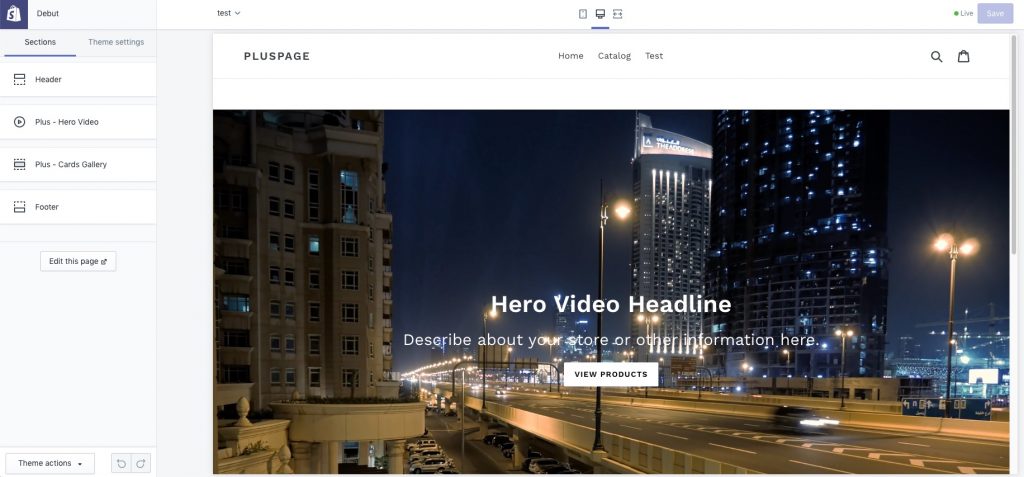This is a low-resolution screenshot of a webpage featuring a prominent photograph that dominates the center of the image. The photo captures a nighttime urban scene under a dark blue sky, showcasing an overpass with a car speeding towards the right. Illuminating the night, the overpass is adorned with streetlights, adding to the urban ambiance.

In the backdrop, two tall skyscrapers, their windows glowing as if people are still working, rise behind the overpass. Further adding to the cityscape, a stadium can be spotted in the lower right corner of the photo.

Centrally positioned within the image, white text reads "Hero Video Headline," followed by a placeholder text "Describe about your store or other information here." Below this, a white rectangle bears the phrase "A few products," indicating an area likely intended for featured products or additional details.